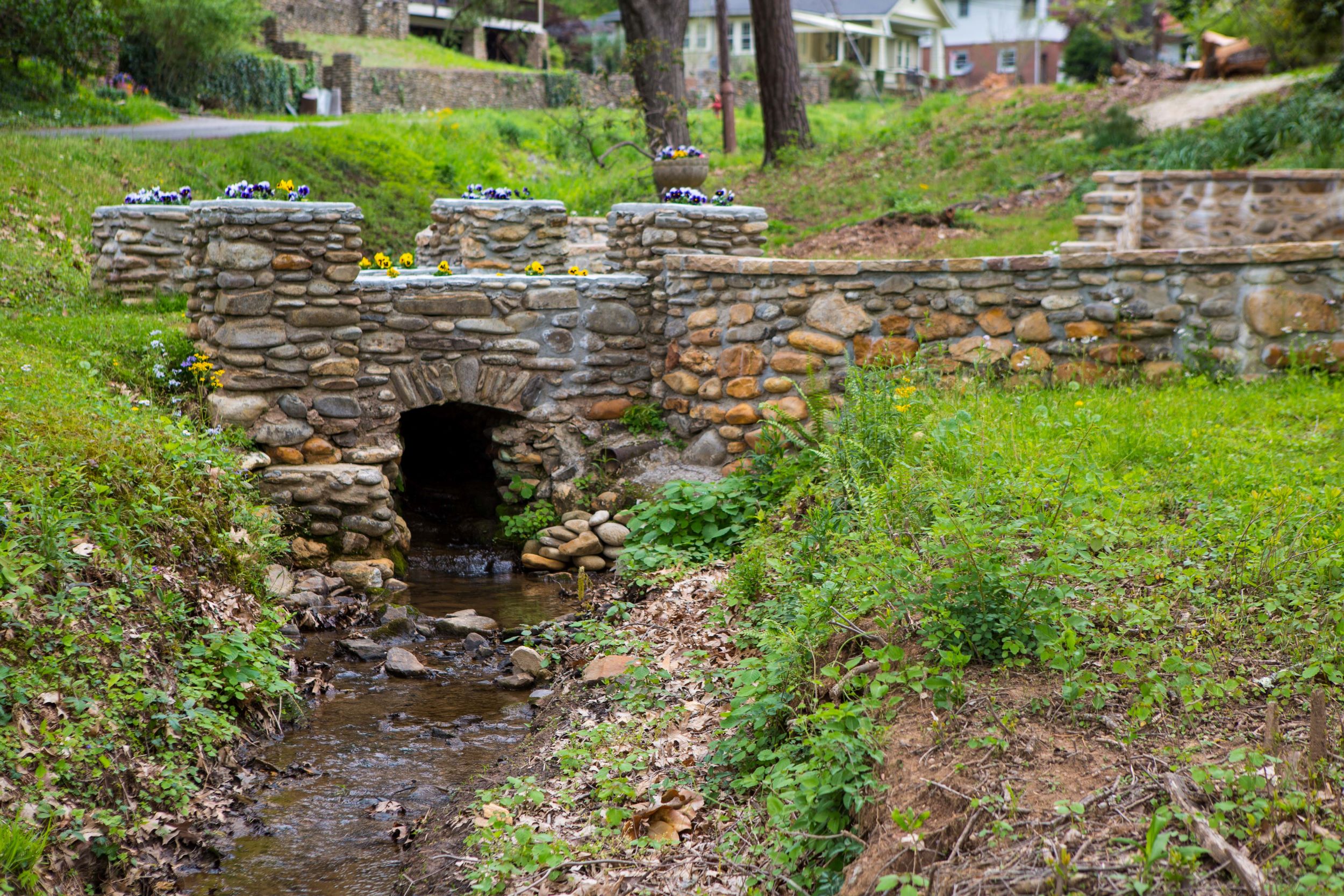In this detailed photograph, we see a quaint, rustic stone bridge made of tan, brown, cream, and gray stones of various sizes and shapes, mostly oval or round. The bridge spans a small brook, featuring four supporting pillars and a lower wall as it crosses the water. On the right, the structure extends into a retaining wall as it meets the land. Surrounding the brook, patches of green grass and well-tended planters displaying purple and yellow flowers adorn the landscape. There are also a few small, potentially breakable animal statues adding charm to the scene. This bridge connects to a sloping paved road, approximately a 30-degree incline, bordered by single-family homes, several of which also feature stone walls, creating a cohesive look throughout the suburban neighborhood. The background highlights these homes and lush greenery, with bushes and trees enhancing the serene, picturesque outdoor setting.